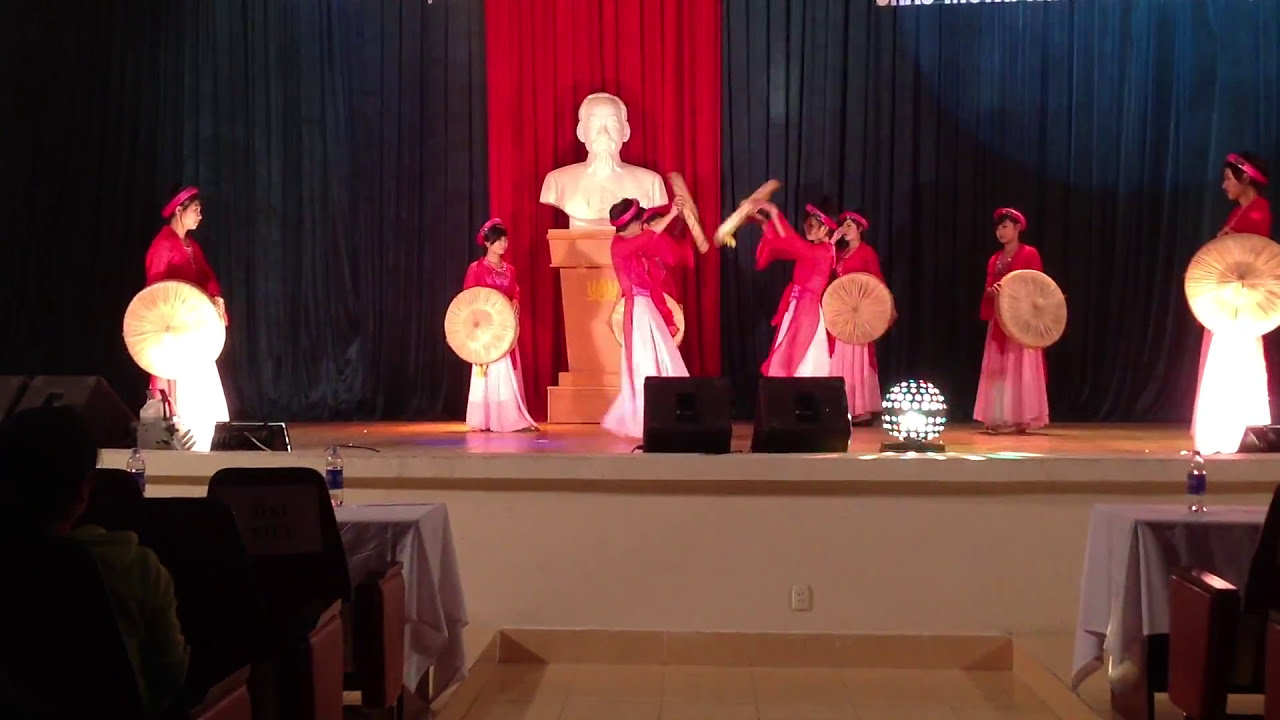The image depicts a detailed scene from an Asian theatrical performance. On stage, eight individuals, who appear to be primarily Asian women, are adorned in red, long-sleeved, flowy shirts or kimonos paired with white skirts. They are holding round objects, likely gray umbrellas or golden shields, which they point towards the audience. Two women in the center are dramatically raising their shields as if pushing them together. Behind the performers stands a prominent white marble statue of a man on a podium, flanked by red curtains directly behind it and black or dark blue curtains to the sides. The stage, viewed from a slightly lower angle, is equipped with various technical elements, including a disco ball-type light, black projecting lights or speakers on either side of it, and additional stage speakers on the ground.